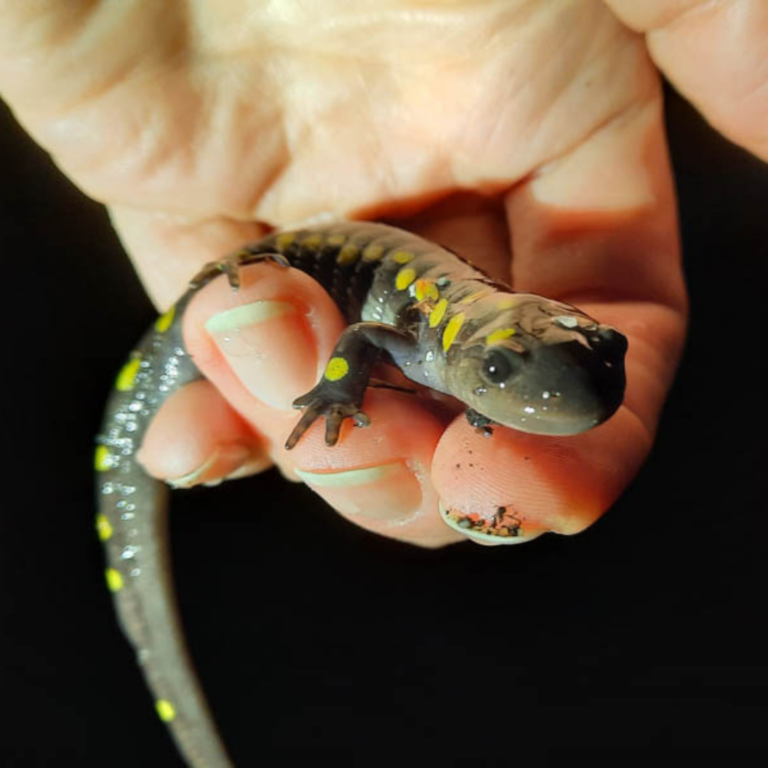The photograph is a close-up color image displaying a small, wet and shiny reptile, either a newt or a salamander, characterized by its dark gray body adorned with yellow dot-like circles lining its back from head to tail and on its legs. The reptile is being held by a person's hand, presumed to be a woman's due to the length of the fingernails, though this could also be a man, as the image of the hand is mostly blurred except for the fingertips. The index finger's fingernail has some dark dirt or crud underneath it. The lizard appears to be gazing directly into the camera, with its head resting on the index finger, its right arm clutching the middle digit, and its right leg positioned on the ring digit of the holder’s hand, while its tail drapes over the edge. The background of the image is entirely black, making the detailed features of the lizard and the hand more pronounced.